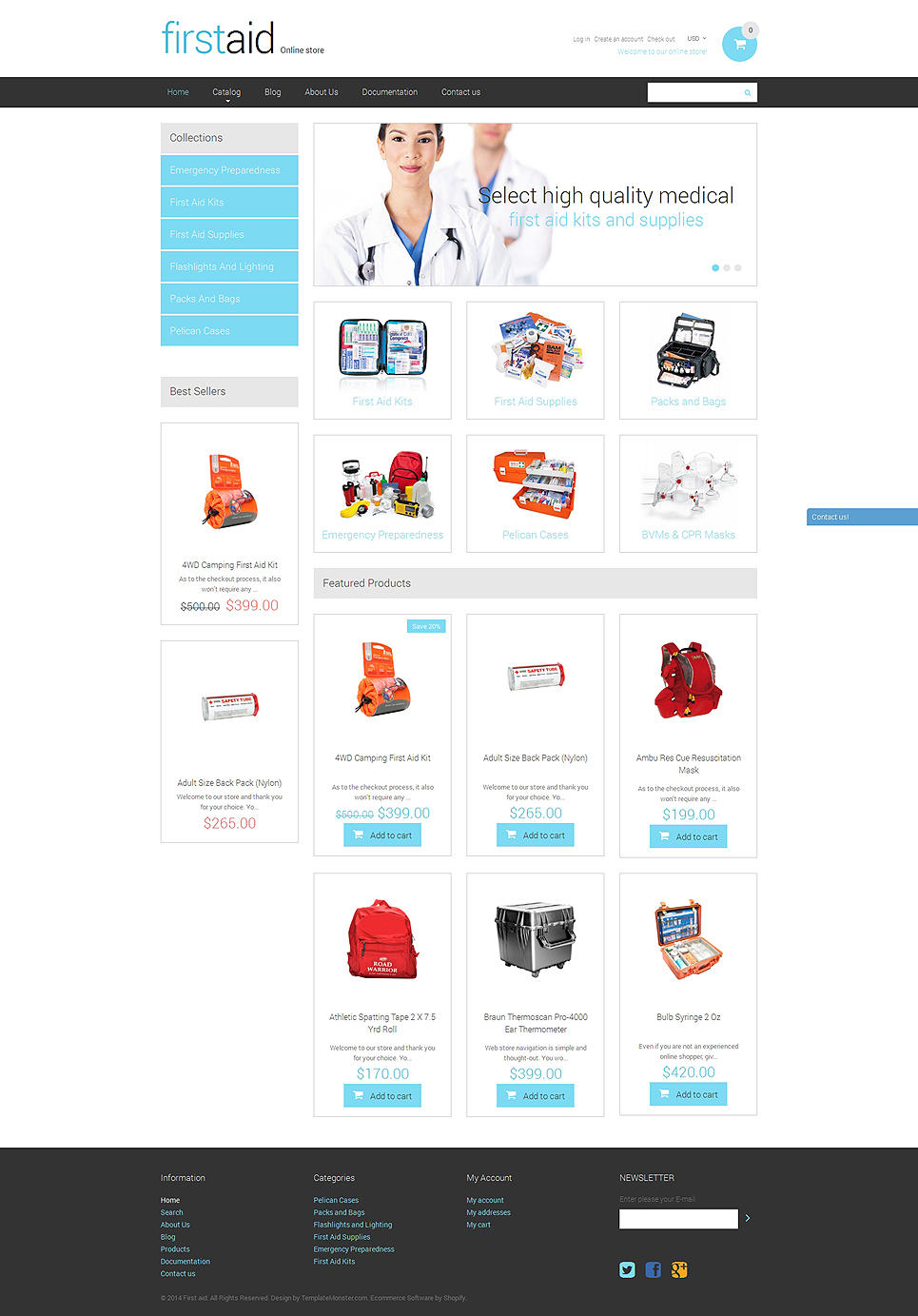The image is a screenshot of a website layout, proportionally about 50% taller than it is wide. 

At the very top, there is a white horizontal banner spanning the width of the site. The banner features the company logo on the left side, which reads "First Aid," with "First" in light blue and "Aid" in black. To the right of the logo, there is a white shopping cart icon enclosed within a light blue circle, though the accompanying text is not readable. 

Below the white banner is a black horizontal navigation bar containing six menu options, which are unreadable due to the small text size. On the right side of this bar is a search box.

Further down, the site includes a left-hand vertical navigation panel slightly indented from the side. This panel lists seven unreadable options. 

The main content banner to the right features an image of two white individuals dressed in lab coats. They appear from the chest up, each wearing faint smiles. Overlaid text on this banner reads: "Select high quality medical first aid kits and supplies," with "Select" and "medical" in black text, and the remaining text in light blue.

Below the main banner is a grid layout displaying various products available for purchase.